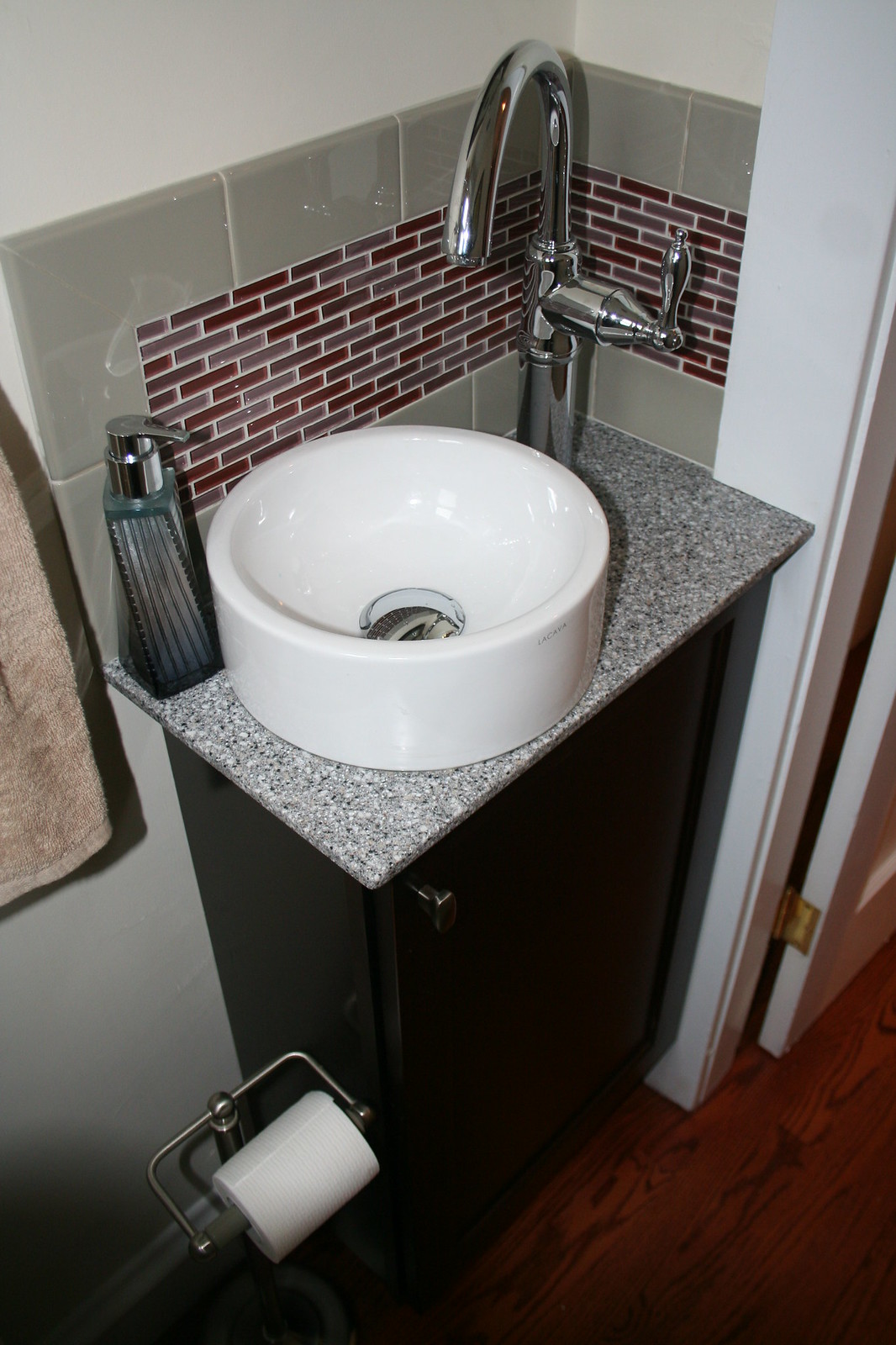The image is a portrait-oriented color photograph capturing the detail of a compact understairs guest toilet in a residential home. Dominating the center of the scene, a round, deep, white ceramic sink is mounted atop a polished granite countertop. The sink, a perfect circle, features a chrome waste cover at its center. Positioned at the back right corner where two walls form a 90-degree angle, a sleek, tall chrome faucet with a single forward-facing lever is installed.

Surrounding the faucet, a small section of tiling adorns both adjacent walls—the tiles extend from a shorter wall aligned with the door frame, continuing along a longer wall that borders the back horizontal side, precisely meeting the granite work surface beneath the sink. Below the counter, a dark, black vanity cupboard is visible although partially shrouded in shadow, hiding its base from view.

To the left of the vanity, a freestanding toilet roll holder made of silver stands upright, holding a white toilet roll. The flooring adds warmth to the space with its cherry-brown mahogany hue, arranged diagonally from the bottom left (8 o'clock) to the top right (2 o'clock) of the image. The wood grain, a rich mix of dark brown and black tones, runs the length of the floor panels, adding texture and depth to the small, stylishly functional area.